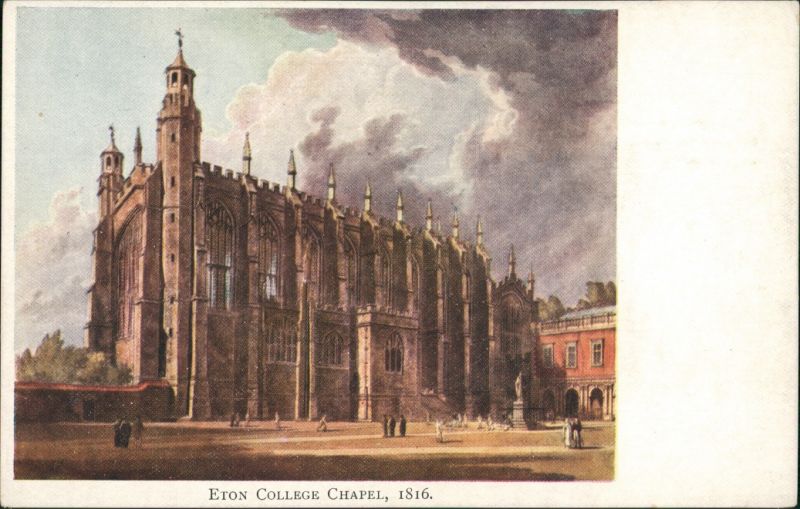The image is a detailed rendering of the Eaton College Chapel in the UK, dated from the year 1816. The painting, positioned slightly to the left within the image border, showcases a sophisticated depiction of the chapel from a ground corner's perspective. The chapel, likely constructed of stone and characterized by its pointed spires, dominates the scene, rising majestically against a backdrop of gray and white clouds. Below the chapel, the courtyard is lively with people milling about on brown dirt paths. Adjacent to the chapel on the right is a smaller building of a different color, adding depth to the scene. In front of the chapel stands a gray statue on a pedestal, presumably of a notable figure. The overall style is reminiscent of historical artwork from a few centuries ago, and beneath the image, bold capital letters read "Eaton College Chapel, 1816." The colors used in the painting, including blue, white, gray, black, red, and various shades of brown, contribute to its antique and lifelike qualities.